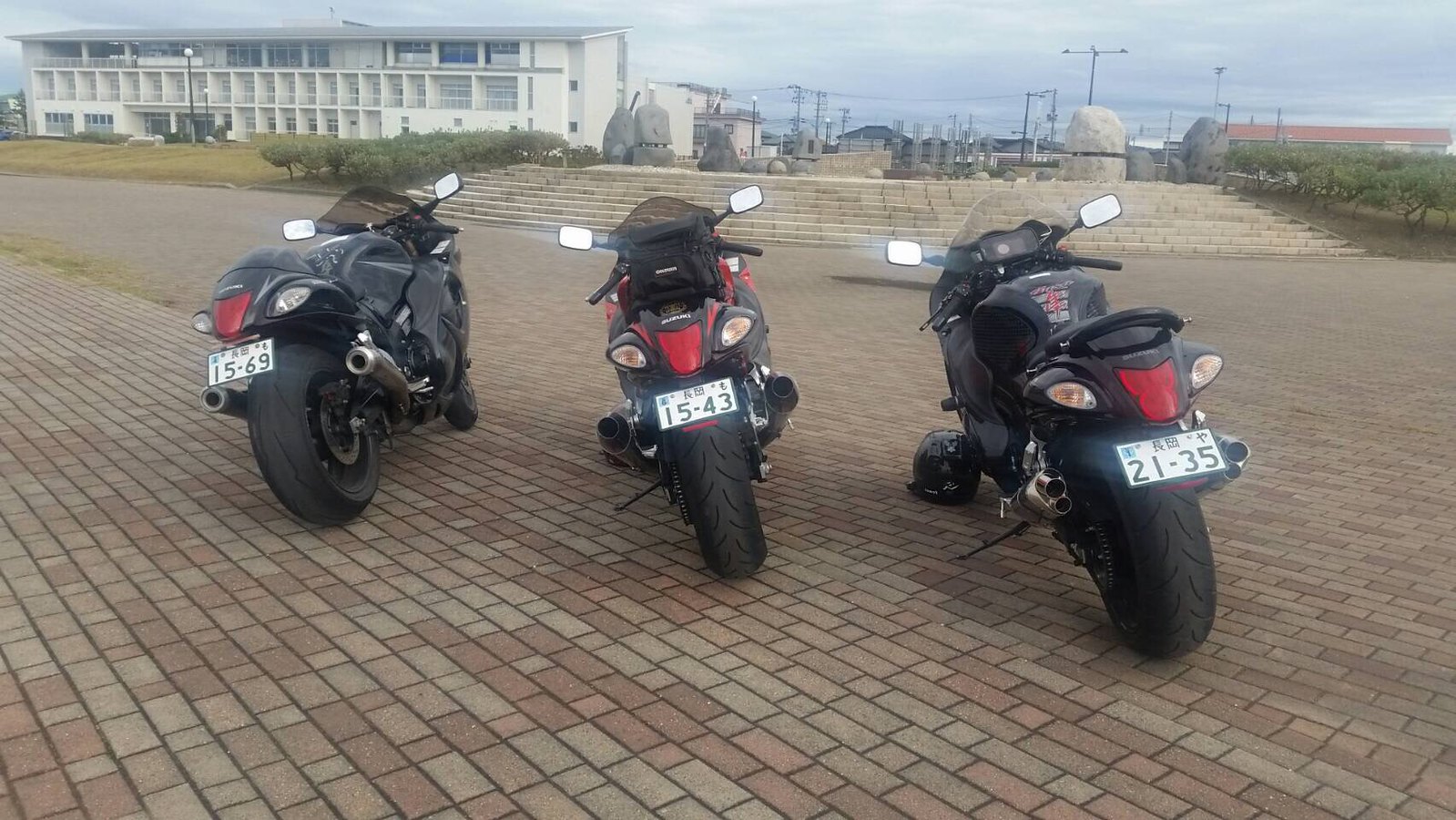In this outdoor image, the sky in the background is a subdued blue with scattered white clouds, and a sense of early morning mist or fog pervades the scene. The right side of the image is lined with several buildings, likely office complexes or hotels, while on the upper left, there's a prominent three-story structure that resembles a motel or condos. Overhead, several telephone or power lines stretch across the sky.

In the foreground, three motorcycles are parked on their kickstands in a circular area paved with reddish-brown and tan cobblestones. The motorcycles, two black and one with a slightly brownish hue, all feature red taillights and uniform white license plates with dark blue alphanumeric characters, pointing to a venue outside the United States. The back tires are closest to the viewer, and the bikes are parked parallel to each other. Adjacent to the paved area are gray steps leading up to the buildings. The overall scene suggests a tranquil setting, possibly near a marina, with the ocean faintly visible beyond the distant buildings.